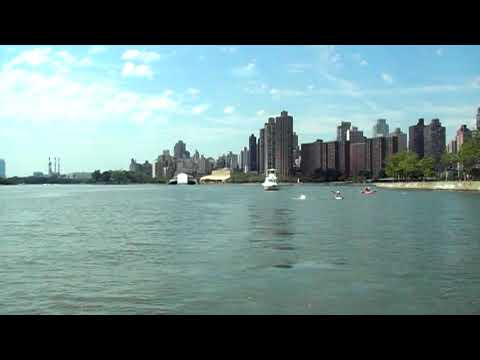The image depicts a large body of water, which could be a lake, bay, or ocean, with distinct urban and natural features surrounding it. In the foreground, two kayakers are visible—one in a bluish kayak and the other in an orangish-red kayak. They are situated slightly to the right of a large, three-tiered white boat that floats prominently in the middle-left section of the image. The water spans the bottom half of the picture and catches hues of blue that mirror the partly cloudy sky. Beyond the water, a tree line can be observed at the shoreline, adding a touch of green to the scene. Further in the background, tall buildings, including both skyscrapers and brownish-gray apartment structures, rise up, forming a dense city skyline. A rock wall also demarcates the transition from land to water. The entire scene suggests an urban waterway, possibly resembling areas like New York City, where natural and metropolitan elements coexist.